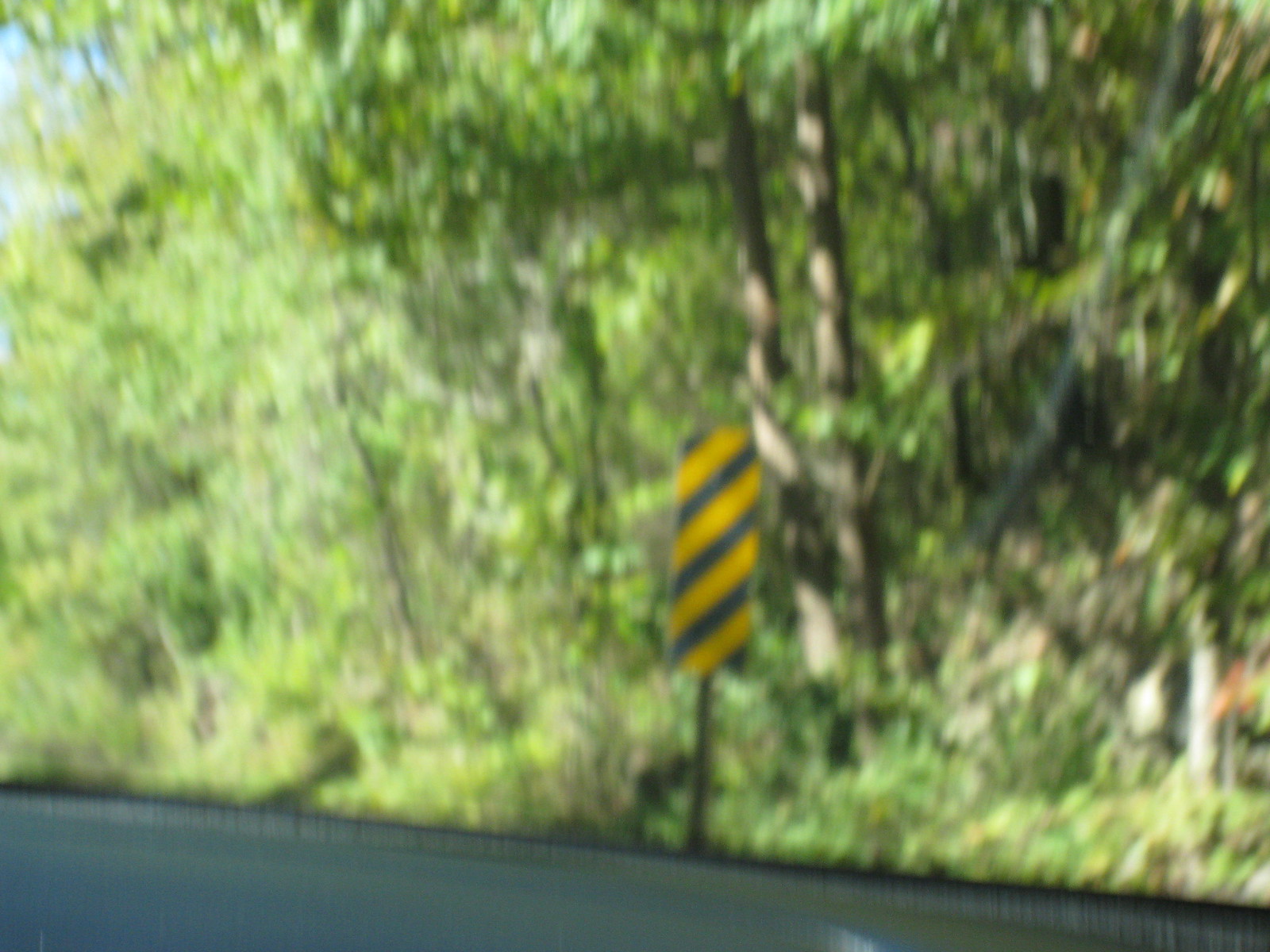A blurry photograph seemingly taken from a moving car captures a cautionary road sign prominently positioned in the front and middle of the frame. The vertical sign features alternating diagonal black and yellow stripes, indicative of a warning for drivers. In the lower part of the image, the car window's edge is visible, reinforcing the notion that the photo was snapped during a drive. Behind the sign, a densely packed cluster of trees with visible trunks suggests it is summertime, contributing to the lush, green backdrop. In the upper left corner, a sliver of sky peeks through, adding to the composition despite the overall blurred nature of the image.